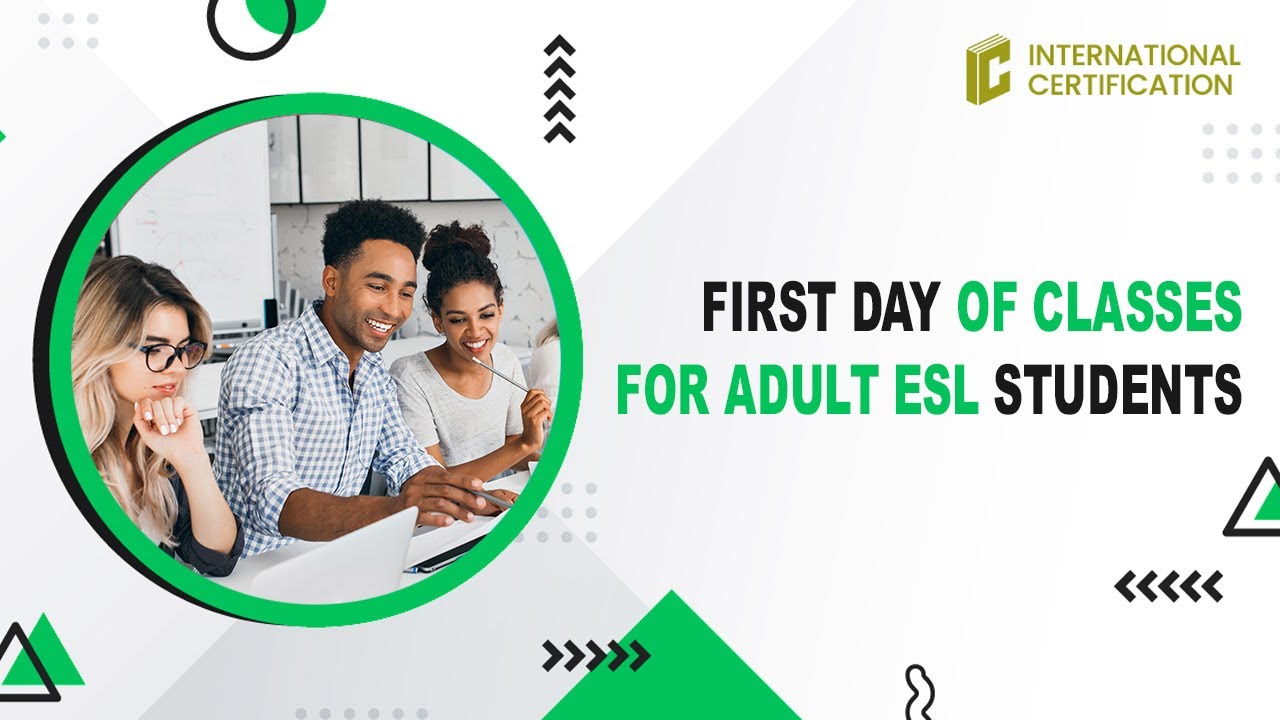This image is an advertisement or a screenshot from a website featuring a white and grey patterned background with circular and triangular detailing, along with black directional arrows. Prominently placed in the center of the image, the text in black and green reads, "First day of classes for adult ESL students." To the upper right corner, there is a yellow "C" logo accompanied by the text "International Certification." 

On the left side of the image's center, there is a large green circle outlined in black. Inside this circle, three individuals are depicted: a woman with blonde hair and glasses, resting her chin on her hand; a man with short black hair in a checkered collared shirt, looking at a computer; and another woman with her hair in a bun, wearing a white shirt and seemingly engaged with what the man is observing. They appear to be in a classroom setting, indicating a collaborative study environment. The intricate design elements and the composition of the image suggest a structured and dynamic educational atmosphere tailored for adult ESL students.